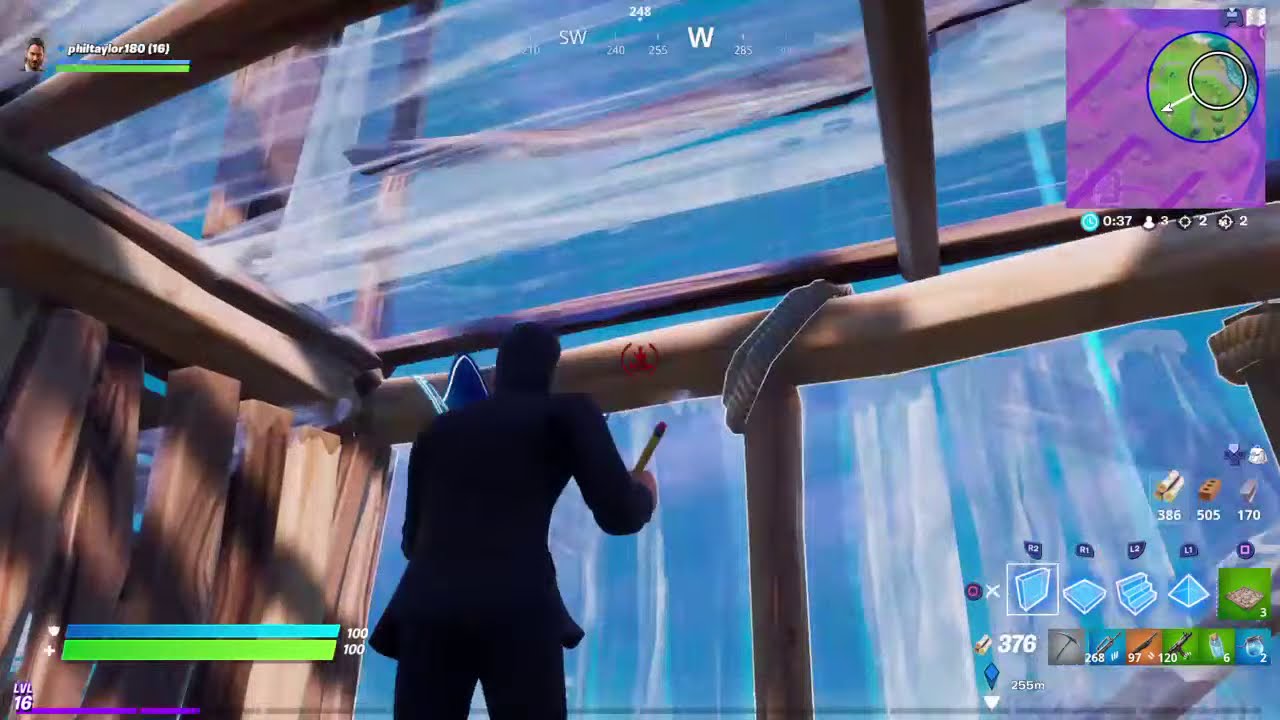In this detailed screenshot from the video game Fortnite, the character is positioned slightly to the left of the frame, showing their back. They are donned in a dark navy blue suit and matching mask, holding a yellow pencil with a pink eraser in their right hand and blueprints that are blue and white. The character is actively constructing a structure composed of wooden elements and vibrant blue glassy areas. The construction features various wooden poles and walls, some encircled by brown ropes, giving it a rudimentary yet functional appearance.

The upper right corner of the screen displays a mini-map with a purple background, a blue circle, and a white circle within the blue. This map highlights grass and street details. In the upper left corner, the navigator indicates cardinal directions (southwest-west 248, 255, 240, 285, and 210) in white letters. The player information shows they are at level 16, with a health bar and a shield bar both at 100%. At the bottom of the screen, there are details about the building materials and available weapons, crucial for gameplay strategy. The display emphasizes the player's current state, fully ready for action within the game's interface.